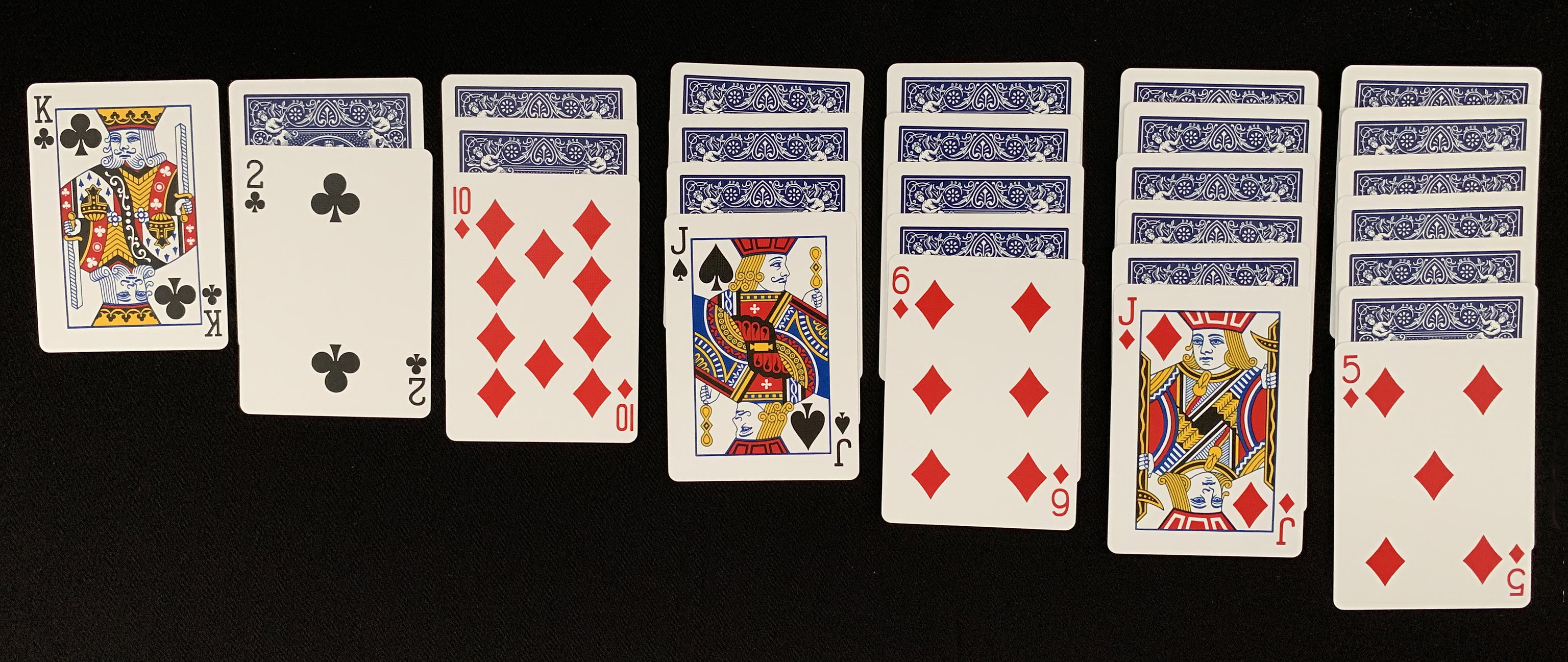The image features a game of solitaire in progress, set against a completely black background. The layout of the cards is as follows, starting from the left side:

- A King of Clubs is positioned first.
- Next to it is a Two of Clubs with one card face down behind it.
- Following that is a Ten of Diamonds with two face-down cards behind it.
- Adjacent to the Ten of Diamonds is a Jack of Spades, under which there are three face-down cards.
- Next in the sequence is a Six of Diamonds, which has four cards face down behind it.
- This is followed by a Jack of Diamonds with five face-down cards behind it.
- The final card visible is a Five of Diamonds, accompanied by six cards face down behind it.

The deck used in this game features a blue and white design. In traditional solitaire rules, players alternate by placing red cards onto black cards and vice versa, ensuring the next card in sequence is one rank lower. For instance, the Ten of Diamonds can be moved onto the Jack of Spades. By doing so, the player would reveal the next face-down card in the Ten of Diamonds’ column, continuing the game by either playing that newly revealed card or drawing from the deck.